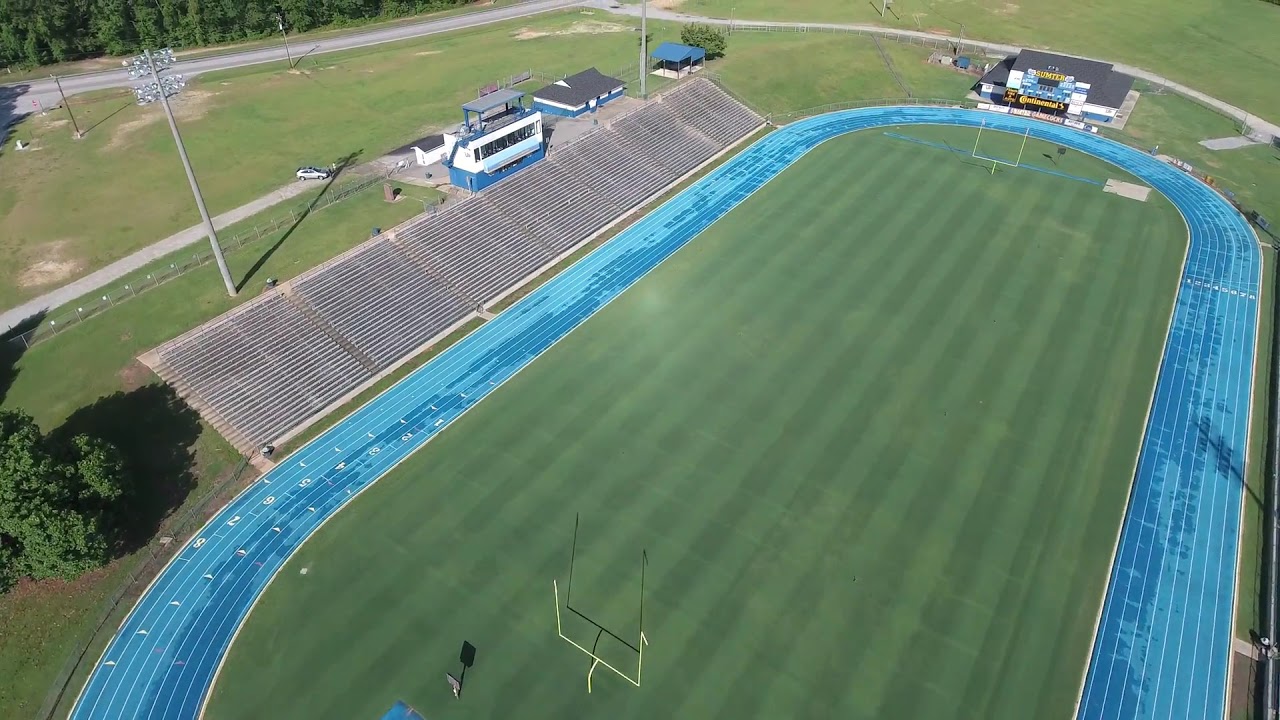This is an aerial view of an American football stadium and its surrounding area. The stadium, rectangular with semicircular ends, features goalposts at each end indicating it's a football field, although it lacks hash marks or yard lines. Encircling the green field is an eight-lane running track, painted in a teal or light blue color, with white lane numbers from one to eight. The stadium is equipped with brown and gray spectator stands, which are currently empty, and a white-sided press box with a blue base situated above them. On one side there's a digital scoreboard, and there are stadium lights positioned beyond the stands. The surrounding area is covered in green grass and includes several buildings, contributing to the stadium's infrastructure.